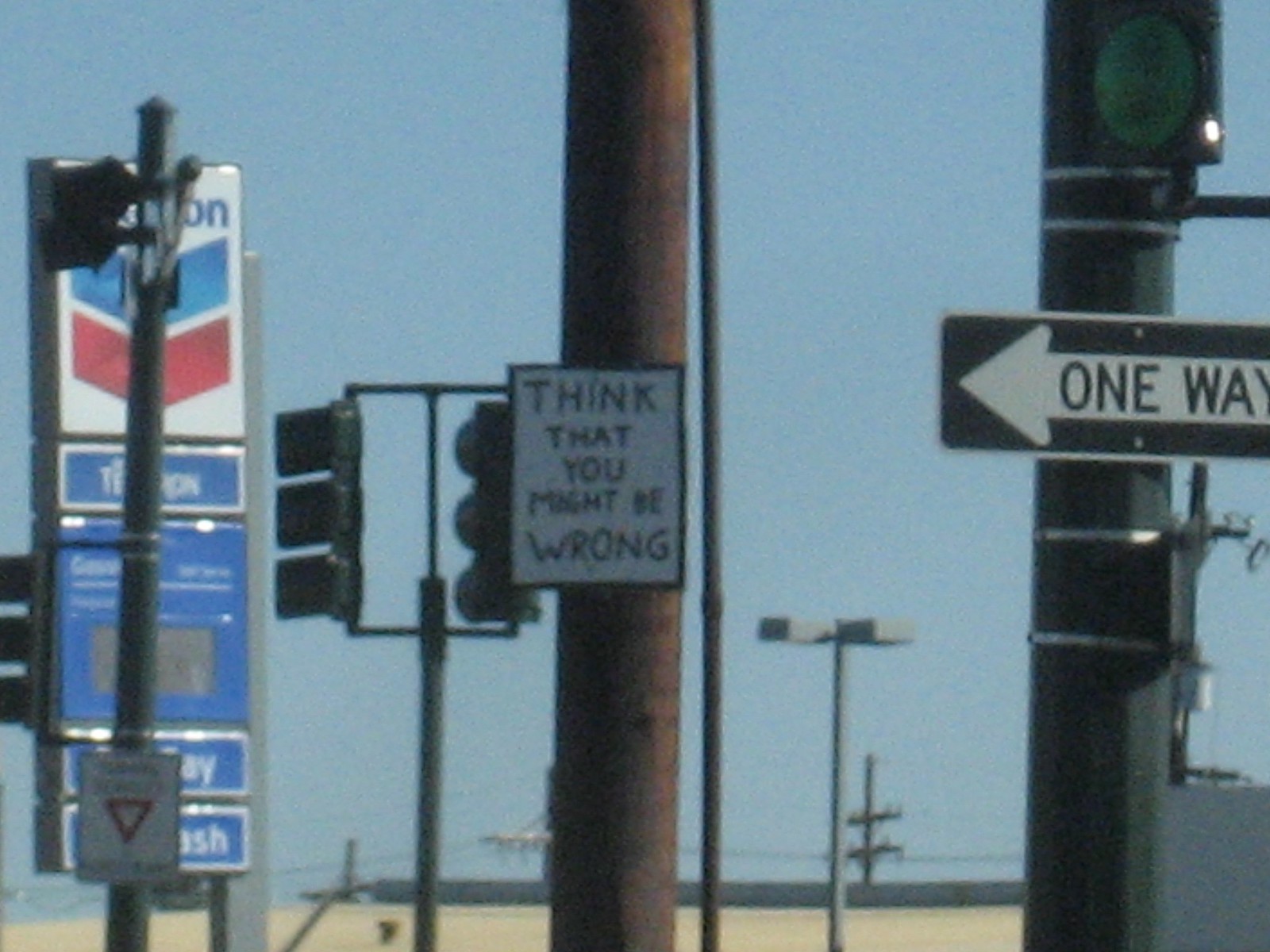The image captures a bustling street intersection under a vivid blue sky, showcasing a variety of traffic signs and signals. Prominently displayed is a Chevron gas station sign, adorned with the brand's distinctive blue and red Chevron symbol atop a white background, though no gas prices are visible. A collection of road signs marks the scene, including a one-way sign with black text and a left-pointing arrow, and a contemplative sign that reads, "Think you might be wrong," mounted on a dark brown pole. Multiple street lights, traffic lights, and power poles populate the area, with clearly visible power lines crisscrossing the background. In the distance, an identifiable yield sign and a glimpse of a tan building's roofline are visible. The bright, sunny day highlights the crispness of the black traffic lights and gray street poles that dot the intersection.